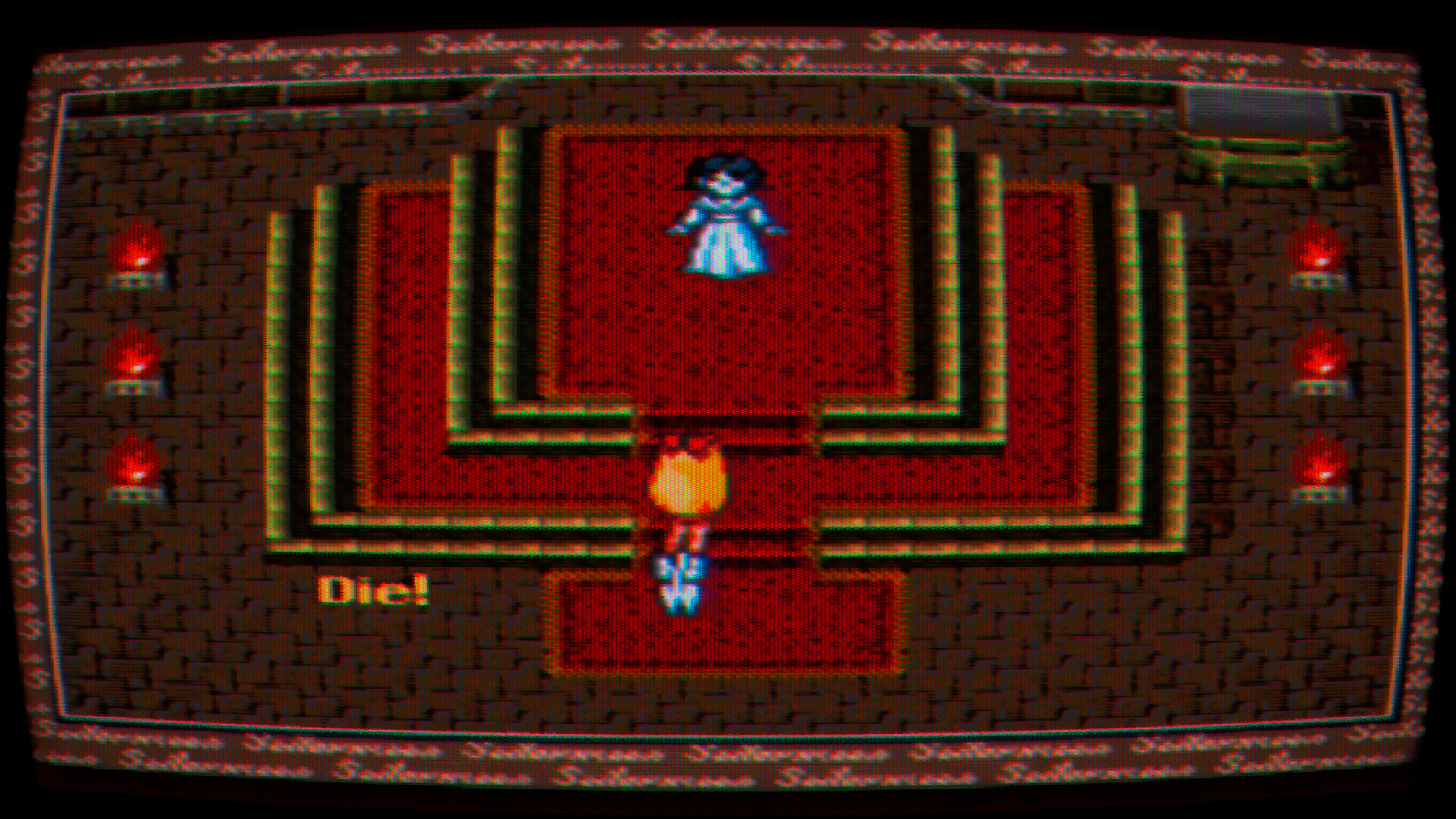A photograph of a vintage video game screen captures a top-down dungeon scene reminiscent of classic Zelda games. The image quality suggests it was taken with a camera rather than a direct screenshot. In the dungeon room, a princess stands elevated on a platform with stairs on either side leading up to her. Strangely, the word "DIE!" is prominently displayed, hinting at an unexpected threat or message, though it’s unclear who the source of the ominous text is.